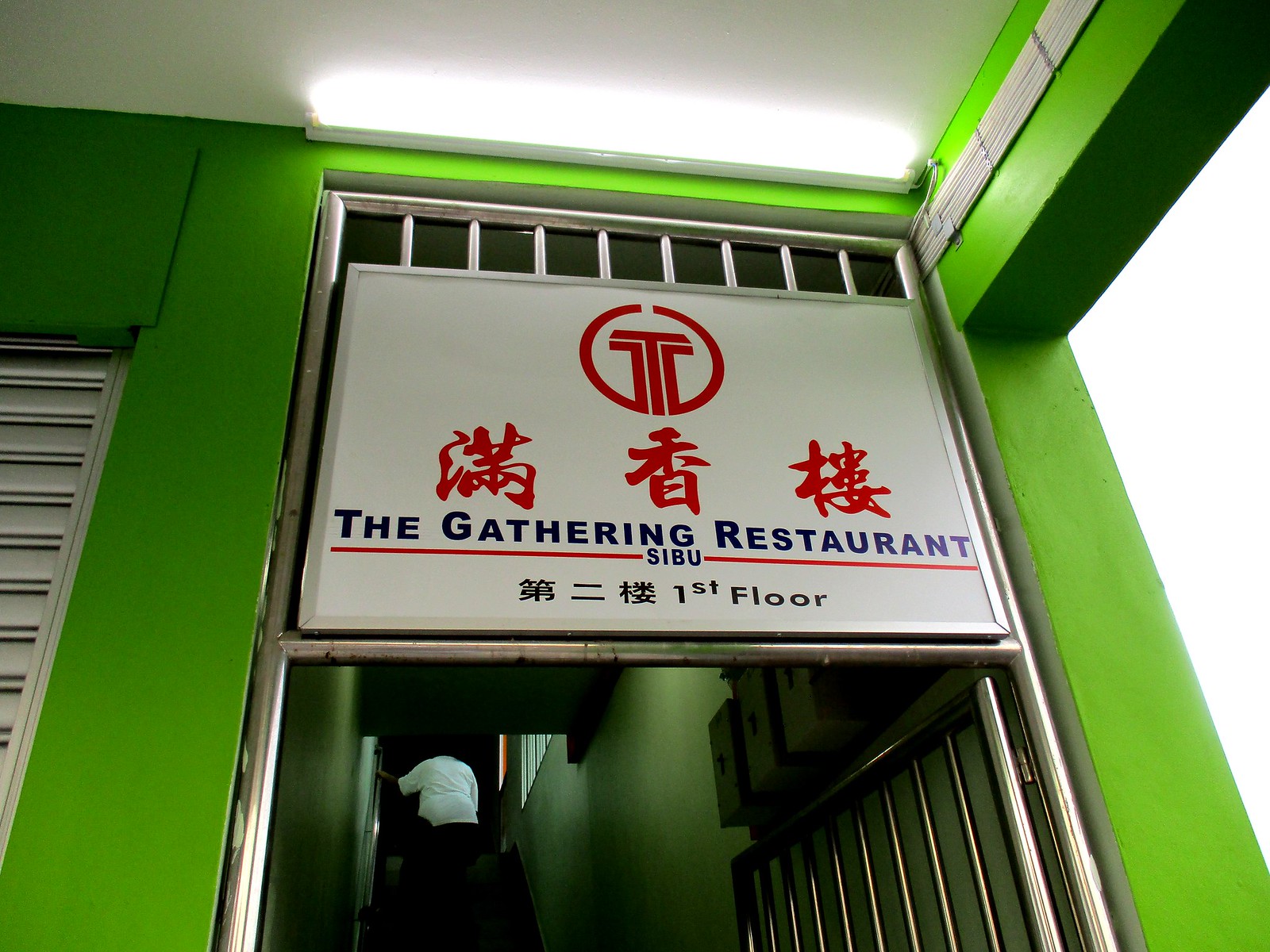The image captures the entrance of a building characterized by a vivid lime green exterior wall. On the left side of the image, a small section of a silver metal gate is visible, leading up to a level flight of stairs flanked by white walls on both sides. Above the entrance, a prominent white signboard displays the name of the restaurant, The Gathering Restaurant, accompanied by a circular T logo and three Chinese characters in red. The sign further indicates the location as Sibu and specifies "The Right First Floor" in both English and Chinese. There's a partially open metal door at the base of the stairs, through which a person in a white shirt can be seen ascending. The destination, The Gathering Restaurant, is situated on the first floor, accessible via these stairs within the lime green walled hallway.